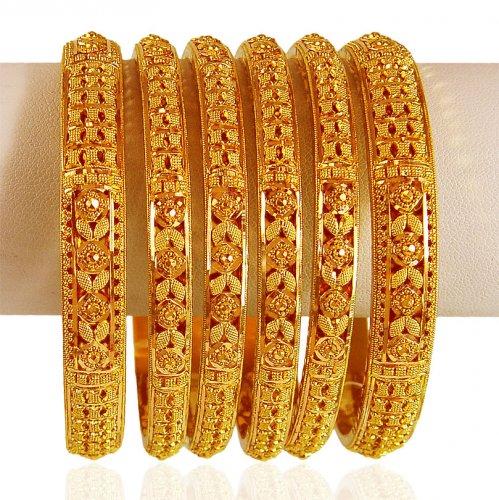This is a detailed close-up image of six intricately designed gold bangle bracelets displayed on a cream-colored leather holder against a white background. The bracelets, which vary in width and pattern, are presented in a way that reflects their ornate craftsmanship. The two on the outer edges are slightly wider than the four centrally placed ones. Each bracelet showcases a beautiful array of carved floral and leaf motifs, along with small embedded gems, squares, dots, and rectangles that add to their elaborate designs. Despite the differences in design, the bracelets appear similar at a glance but upon closer inspection, reveal their unique details. The vivid reflection at the bottom of the image emphasizes the pristine white surface on which the display rests, enhancing the overall elegance of the scene.